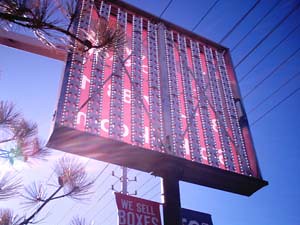Shot outdoors from a ground-level perspective, this photograph captures the underside of an illuminated sign against a clear blue sky. The focal point of the image is the backside of the sign, which is mounted on a large, round metal pole. Vertical strips of lights run across the back of the sign, revealing its intricate metal skeleton framework. Through these slats, one can glimpse a red, transparent plastic face that would glow vividly when the sign is illuminated. The background is accentuated by the silhouettes of tree branches adorned with needles instead of leaves, adding a natural touch to the industrial scene. Additionally, telephone or electrical wires crisscross the sky, integrating elements of urban infrastructure into the composition.